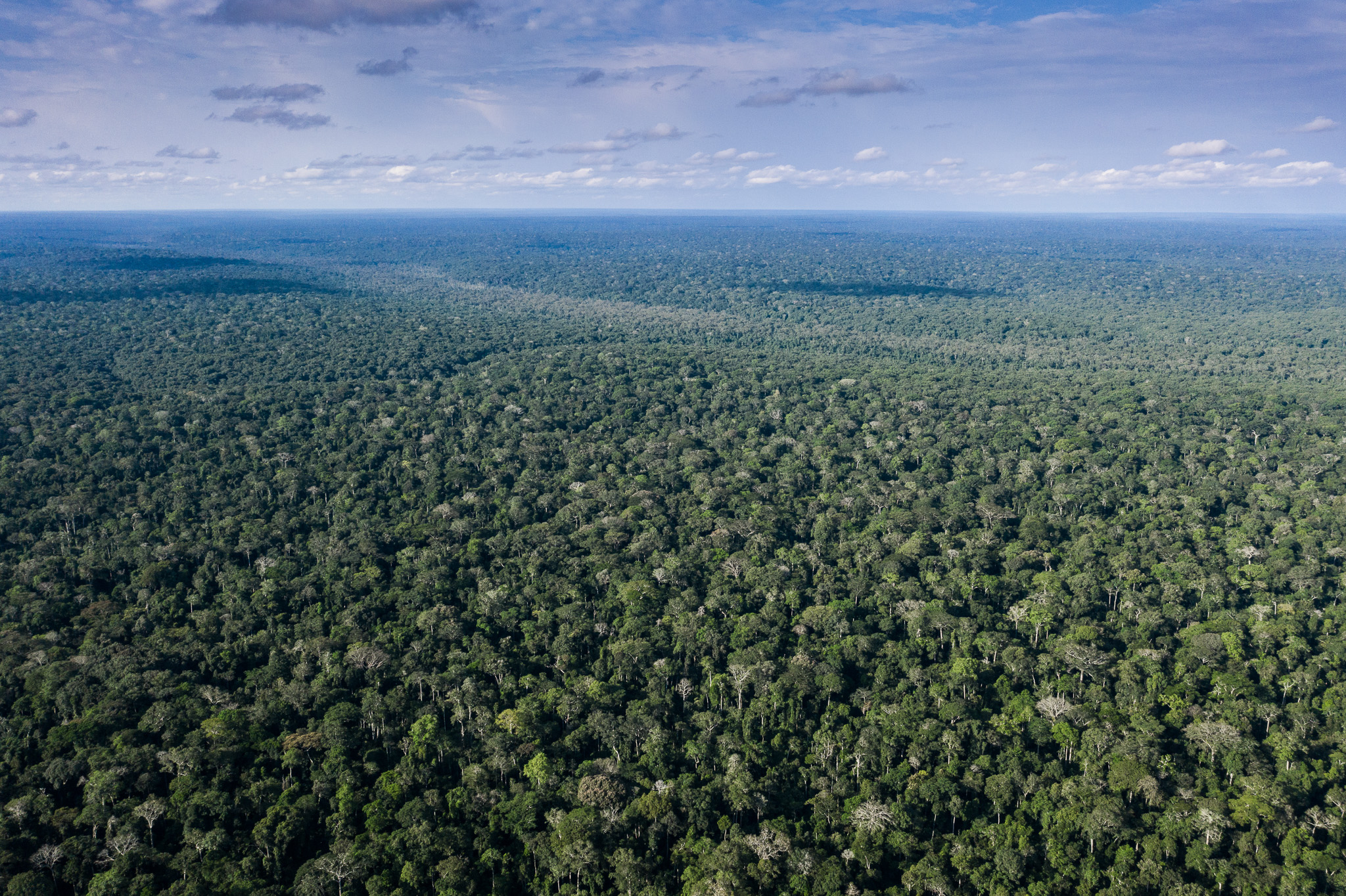This image is an aerial photograph capturing an extensive forest that stretches as far as the eye can see. The landscape is predominantly composed of green treetops, interspersed with a few that are either leafless or dead, identifiable by their differing hues. The photograph depicts a flat terrain, devoid of any signs of human civilization such as roads, homes, industrial structures, or power lines. Shadows cast by clouds are visible on the forest canopy, adding texture to the sea of green. In the distance, the verdant expanse gradually transitions to a bluish haze as it meets the horizon. The sky above is partly cloudy, with layers of white and blue clouds, and patches of blue sky peeking through. The overall scene conveys a sense of untouched wilderness, with nothing but trees and the vast sky above.